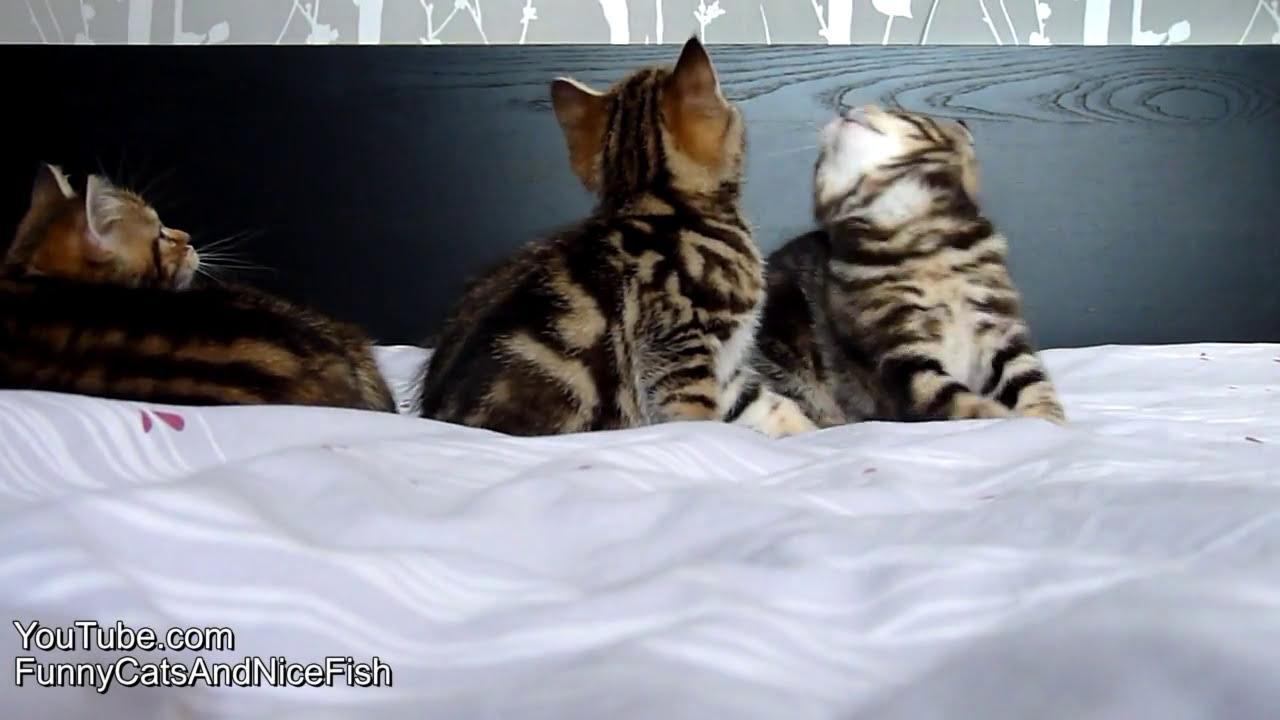This image features three adorable kittens, likely of an exotic breed such as Bengal, lounging on a bed. The bed has an elegant black wooden headboard, set against a backdrop of gray and white floral wallpaper. The bedding is predominantly white with hints of gray and possibly pink accents, forming a subtle, delicate pattern. In the lower right-hand corner, there's text that reads "youtube.com Funny Cats and Nice Fish," indicating this is a still from a YouTube video. The kittens, colored in shades of black, tan, brown, and white, are all intently looking upwards, capturing a moment of shared curiosity. One kitten is poised to pounce, another stands on all fours, and the third lies down, all fixated on something above. Despite not being a professional picture, the composition and the detailed, charming demeanor of the kittens make it an endearing capture.